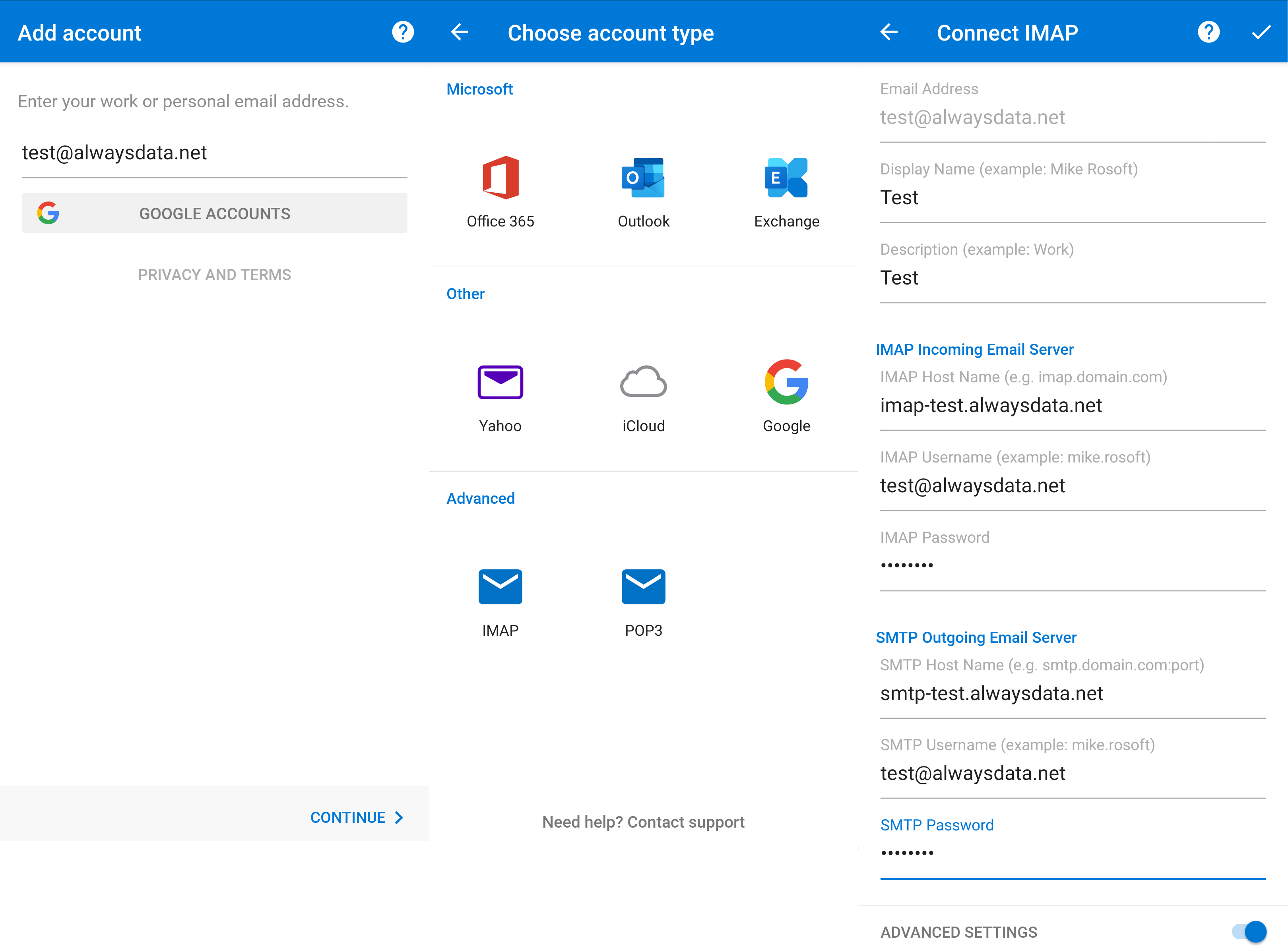A screenshot displays the interface for adding an IMAP account for email synchronization. The page includes various options for selecting email service providers, including "Microsoft Office 365," "Outlook," "Exchange," "Yahoo," "iCloud," and "Google." Additionally, users can opt to set up "Advanced IMAP" and "POP3." 

There are multiple sections visible in the screenshot:
- "Test always data NAT" appears as a default entry.
- An area labeled "Google accounts, privacy and terms continue" suggests that privacy settings and terms of service are in focus.
- For IMAP configuration, fields are populated with server details: 
  - "IMAP incoming email server" is set to "imap.test.alwaysdata.net."
  - The username is given as "test@alwaysdata.net."
  - The user is prompted to enter a password.
- For SMTP configuration, fields are similarly populated: 
  - "SMTP outgoing email server" is addressed as "smtp.test.alwaysdata.net."
  - The SMTP username is also "test@alwaysdata.net."
- An "Advanced settings" toggle is turned on.

Additionally, options like "Need help?" and "Contact support" are available for user assistance. The interface is user-friendly with clear distinctions for server settings and login credentials to ensure proper email account integration.